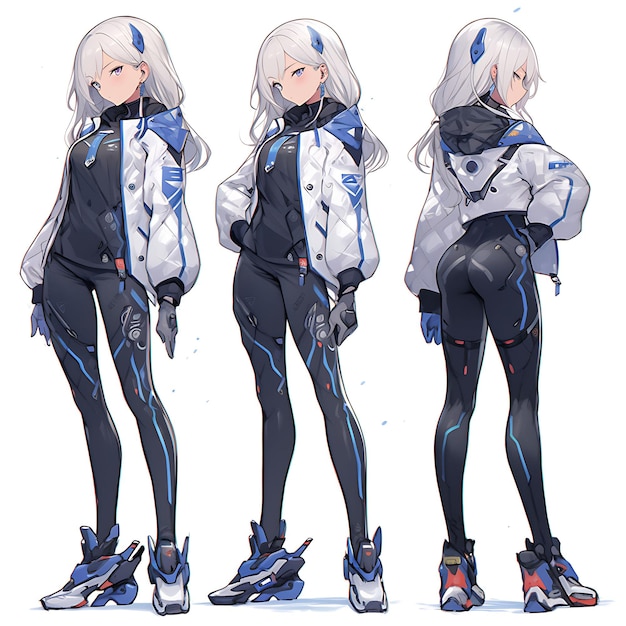This anime-style illustration features three different poses of the same character, showcasing a detailed and futuristic aesthetic. The character stands on the left facing left with her arms against her sides and her head slightly tilted. In the middle pose, she has one hand in her pocket, and the other at her side, with her head tilted downwards. On the right, the character is viewed from the back, revealing her body and showcasing that the jacket doesn't cover her backside. She has long white hair adorned with a small blue clip, light-colored eyes, and distinct facial features that notably lack a visible mouth and nose, focusing instead on large, expressive eyes. Her ensemble includes a snug black top, tight black pants with blue stripes on the sides, and a white, slightly puffy jacket. Completing her futuristic look are her unique shoes, which appear robotic or Gundam-inspired, suggesting a potential transformation ability or advanced technological features.